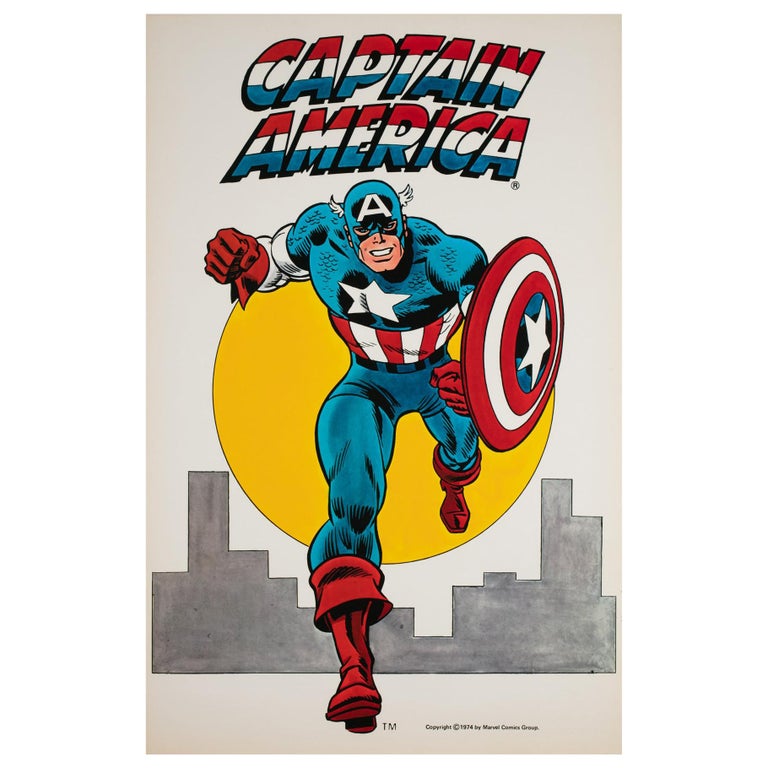This detailed poster or cut-out page from a comic magazine showcases the iconic figure of Captain America in an intense action scene. At the top of the poster, the name "Captain America" is prominently displayed in a stylized red, white, and blue font, reminiscent of the American flag. Below the title, Captain America is depicted sprinting directly toward the viewer with his shield and fist raised, his face etched with determination. His costume features the patriotic colors of blue, white, and red, complete with a white star on his chest, red boots, and blue tights. His distinct headpiece includes wings on either side and a large letter 'A' on his forehead. Captain America wields his indestructible shield, which bears the iconic red, white, and blue concentric circles surrounding a central white star. The background reveals a cityscape silhouette and a circular yellow object, likely symbolizing the sun, from which he appears to be running away. The detailed rendering portrays Captain America's super strength and speed, capturing the essence of this beloved fictional superhero.